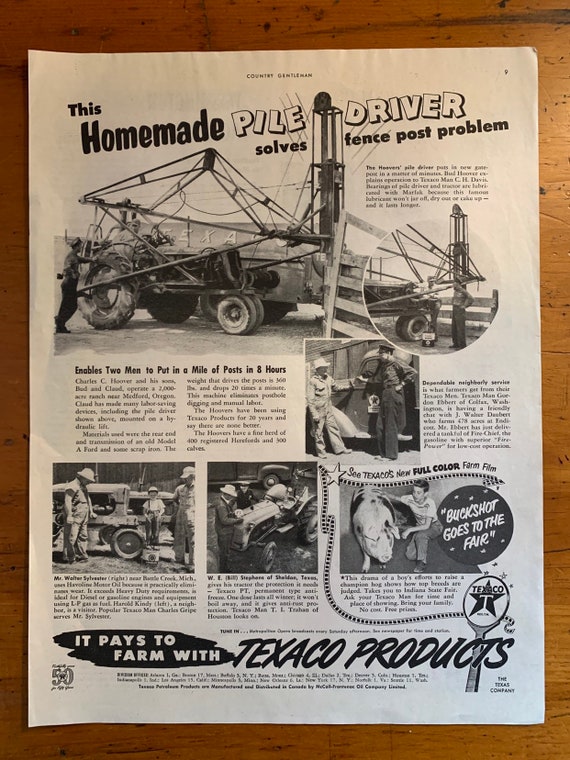The image appears to be a detailed, full-page advertisement from a vintage magazine or newspaper, displaying the page number nine at the top right. At the very top of the page, faint text reads "Country Gentleman." The main headline boldly states, "This homemade pile driver solves fence post problem." The advertisement is entirely in black and white and printed on a piece of paper placed on a brown wooden surface.

There are several photographs spread across the page. The top section prominently shows an old tractor equipped with a pile driver, surrounded by individuals observing its operation. The images depict the pile driver in action, driving down fence posts. Below these photographs, small black text provides detailed descriptions and captions for each image. 

Towards the lower part of the page, there are three additional images: one shows three people standing around a tractor, the center image features a single individual with the tractor, and the rightmost image captures a young man with a pig and a darkened gray circle bearing the caption, "Buckshot goes to the fair."

Further down, in bold white text on a black paint stroke, the slogan reads, "It pays to farm with Texaco products," with "Texaco" prominently highlighted in larger black lettering. The bottom right corner of the page showcases a Texaco logo, and on the bottom left, partially hidden smaller writing including a possible number "50."